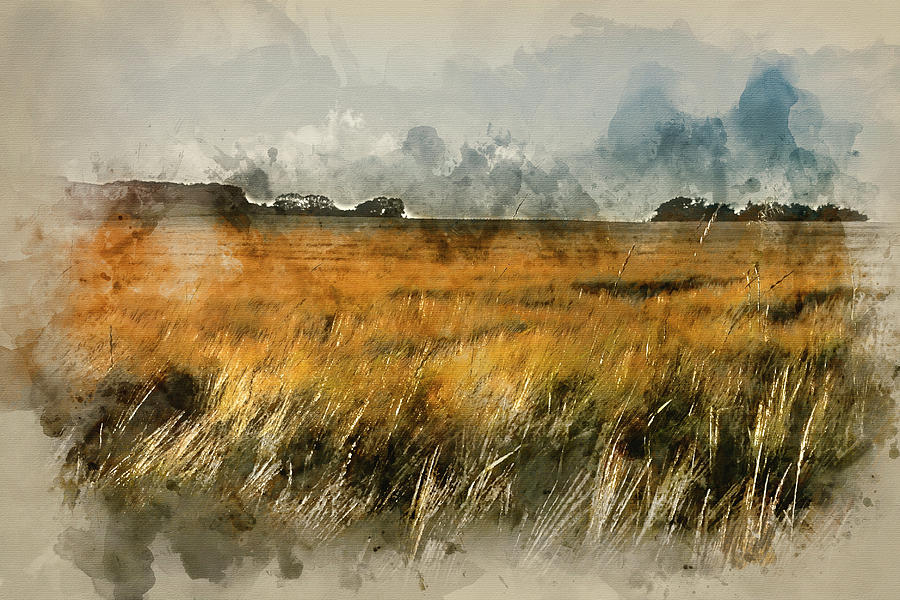This image is a detailed watercolor painting or print, depicting an expansive grassy plain that sways gently to the right. The grass is rendered in hues of yellow, brown, orange, and white, extending back toward the horizon. The background features a mesa visible to the top left, and the horizon is lined with faint outlines of trees. On the far right, there is another cluster of trees. The sky is portrayed in blues with varying intensities, some areas darker possibly to imply impending storm clouds. White clouds stretch in a line from left to right across the sky. The entire edge of the painting is blotted with colors, with grays at the bottom gradually transitioning to blues at the top. The painting includes no text, people, or animals, and the artist's name and vintage are not visible.